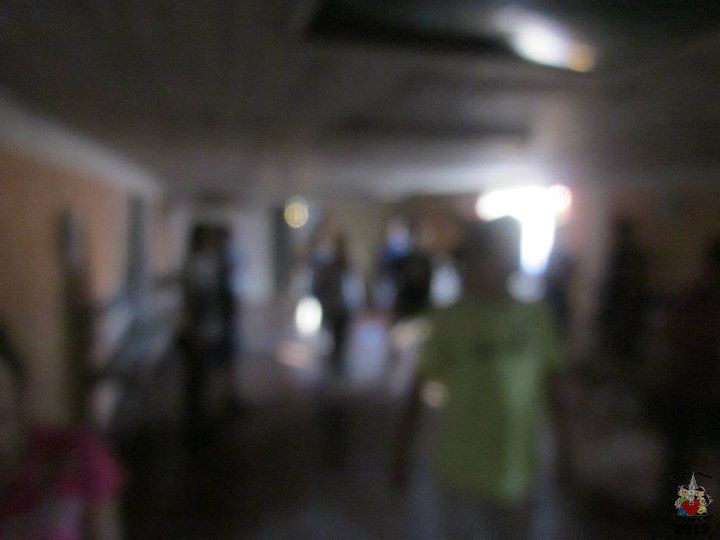The extremely blurry image appears to depict an indoor setting that could be a gym, garage, or store. The room is dimly lit with light shining in from an open door at the back, forming an almost upside-down L shape. The space features a brown wall with a gray border and possibly a bench in front of it. The floor seems to be grayish, and there are white trimmings at the top left and bottom left corners. Around five or six people are visible, though they appear as black figures or blurs. In the foreground, one person wearing a lime green shirt and gray pants stands out, especially to the right of center, moving towards the viewer. To the left, another figure in a pink short-sleeved shirt can be seen, their head outlined clearly. There might be another person in a yellow shirt as well. The overall scene is quite indistinct, almost as if viewed through an underwater lens, making precise details hard to discern.